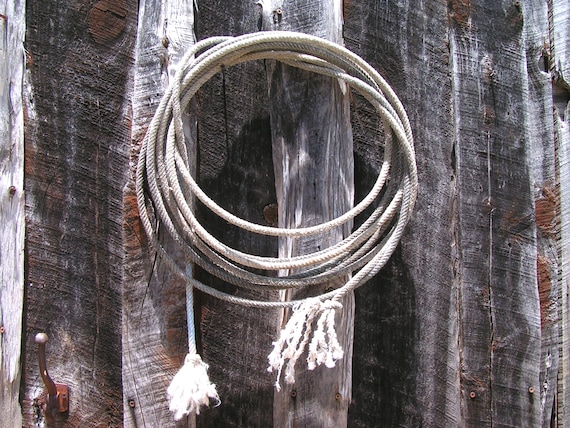This image depicts a coiled, frayed rope organized in a circle, hanging on a very aged and weathered wooden wall or fence. The rope, originally white, now appears grayish-white with signs of wear and dirt, and its ends are noticeably frayed. The wooden structure, possibly part of a barn, is severely weathered, displaying shades of gray, light and dark, with some rusty brown sections. The wood planks and beams are old and irregular, with visible knots, striations, and worn patches, suggesting they were hand-hewn. In the bottom left corner, there is a very rusty nail or hook, accompanied by a couple of screws driven into the planks. Additionally, slight chunks of red can be seen where non-rotted wood peeks through the gray. The overall scene radiates a rustic and historic charm, underscored by the decrepit state of the materials.